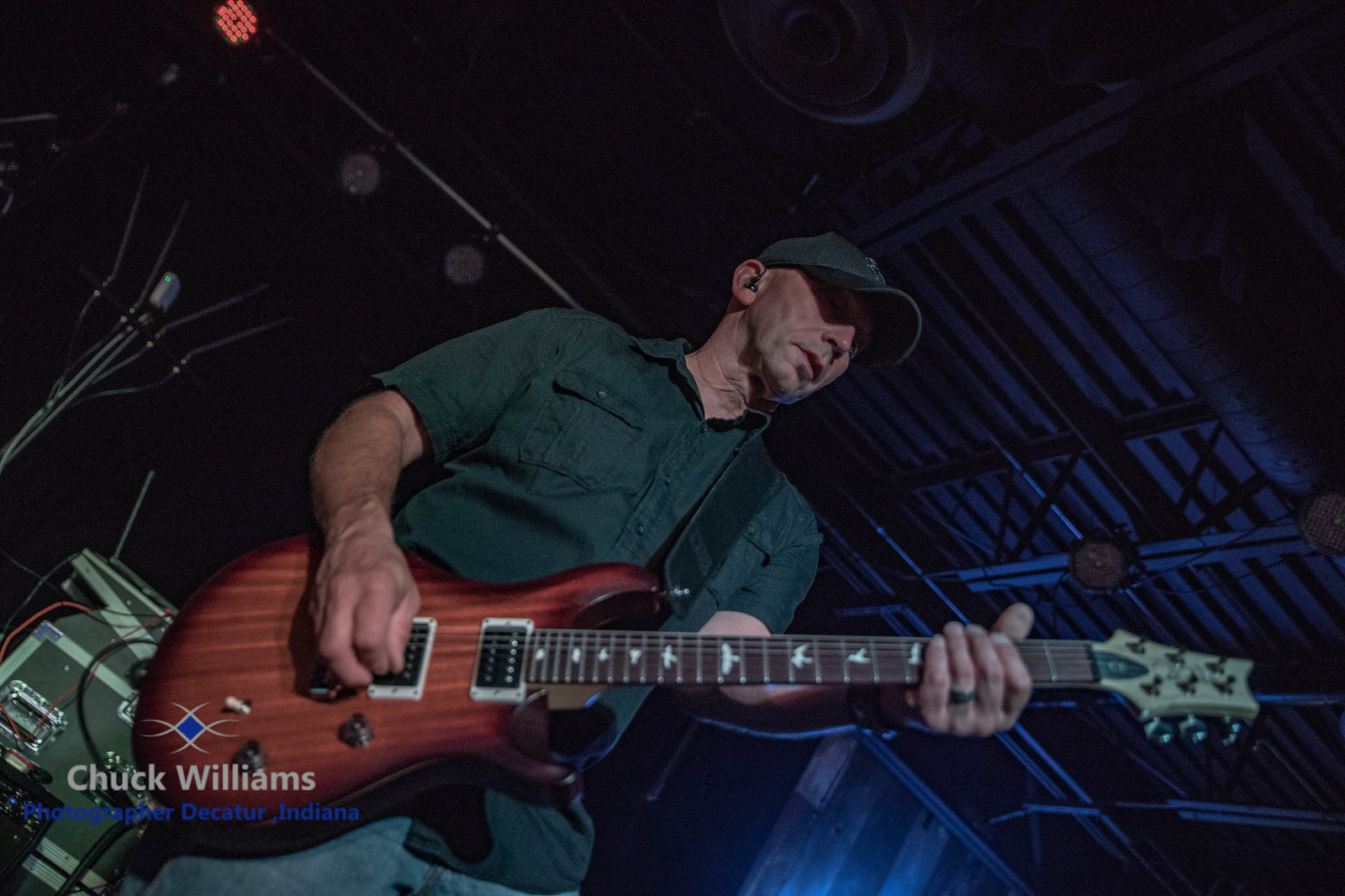In this image, a white man is captured mid-performance playing a six-string electric guitar on a dimly lit stage, likely at a club or concert hall. The shot, taken from below, accentuates the dark surroundings highlighted by subtle blue and red lighting. Wearing a forest green short-sleeve button-up shirt, blue jeans, and a dark green or black hat, he strums the guitar with his right hand while the fretboard is adorned with white bird decals. The guitar itself boasts a dark wooden color. Behind him, to the left, an amplifier is visible, suggesting the setup is for a live performance. A large crate, possibly for equipment, along with an unusual light fixture, can be seen in the background. In the lower-left corner, the photograph is credited to Chuck Williams, Decatur, Indiana, in white text.